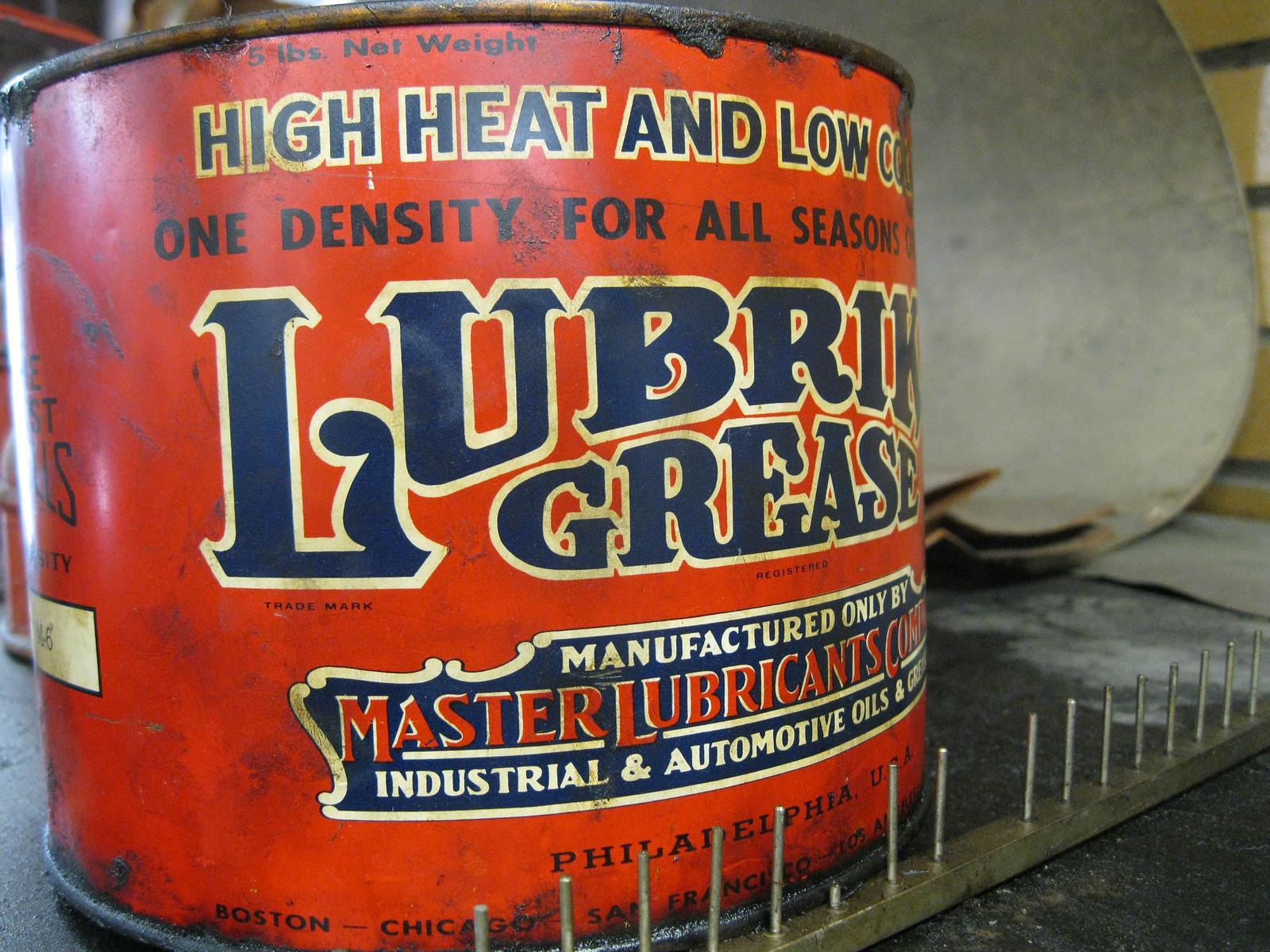The photograph depicts an old, rusted 5-gallon can of Lubrik grease lying on a rough, cemented surface, possibly in the interior of a garage. The can, predominantly displaying a blue font with a white outline, partially reads at the top, "high heat and low...," further obscured as it wraps around the can. The central text declares, "One density for all seasons," with additional labeling reading, "Lubrik Grease, manufactured only by Master Lubricants Industrial and Automotive Oils, Philadelphia, USA." Below, smaller print lists various city names including Chicago, Boston, and San Francisco, among others. A metal rod with spikes extends in front of the can, suggesting a storage function or protective barrier. In the background, the dense, orange-hued setting hints at typical garage clutter, with an ambiguous, round metallic object to the right, possibly a bucket or a large dish. The scene is illuminated with neutral tones, incorporating shades of red, blue, white, brown, tan, and gray, indicating a well-lit, indoor environment.